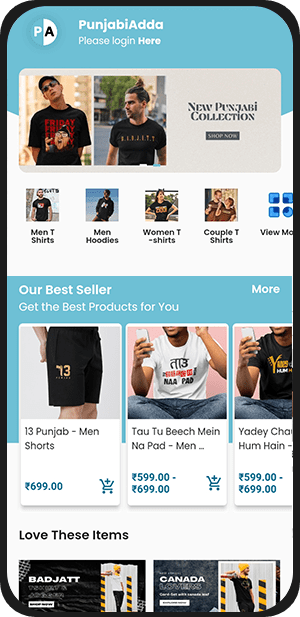This image showcases a detailed mockup of a shopping app displayed on a smartphone. The mockup does not depict an actual phone but rather a conceptual representation, emphasized by its black border. Within this border, the primary colors are sky blue and white, providing a clean and modern interface.

At the top of the screen, there is a logo which appears to be a circle divided into two halves: the left half is light blue with a white "P," and the right half is white with a black "A." To the right of the logo, there is a word, likely the company name, which may be difficult to pronounce, followed by the text "Please log in here" in white.

Beneath the header, the app features multiple thumbnails of male models showcasing various clothing items such as graphic tees and shorts. These images introduce the men's clothing section. Following this, there are clickable categories for various types of apparel, including "Men's T-Shirts," "Men's Hoodies," "Women's T-Shirts," "Couple T-Shirts," and a "View More" option, each represented by a model in relevant attire.

Further down, a section labeled "Our Bestsellers" highlights popular products with the tagline "Get the best products for you." This section showcases three thumbnails: a pair of men's shorts priced at $6.99, and two shirts modeled by the same man, priced between $5.99 and $6.99.

At the bottom of the mockup, there are two clickable sections for more curated collections. The first section is not clearly named, while the second one says "Canada" followed by "something," each featuring the same model in different outfits.

Overall, the image effectively conveys the layout and visual appeal of the shopping app, targeting a stylish and user-friendly shopping experience.